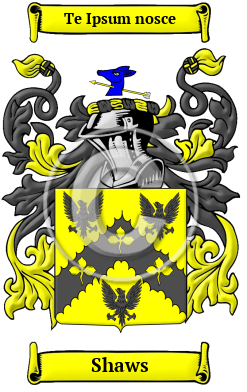The image depicts a meticulously designed coat of arms against a white background. At the top, a bright yellow banner rolls up at the edges, inscribed with the Latin phrase "Te Ipsum Nascae" in black letters. An identical yellow banner at the bottom bears the family name "Shaws." The central emblem features a prominent yellow shield adorned with an inverted black V, highlighted by three yellow clovers. Perched on and around the shield are three black eagles, two on the upper banner, and one below. The centerpiece of the coat of arms is a striking blue deer's head punctured by an arrow, positioned above a traditional knight's helmet. Surrounding the shield and helmet are elaborate black and yellow tassels and swirls, adding a sense of grandeur and intricacy to the design.